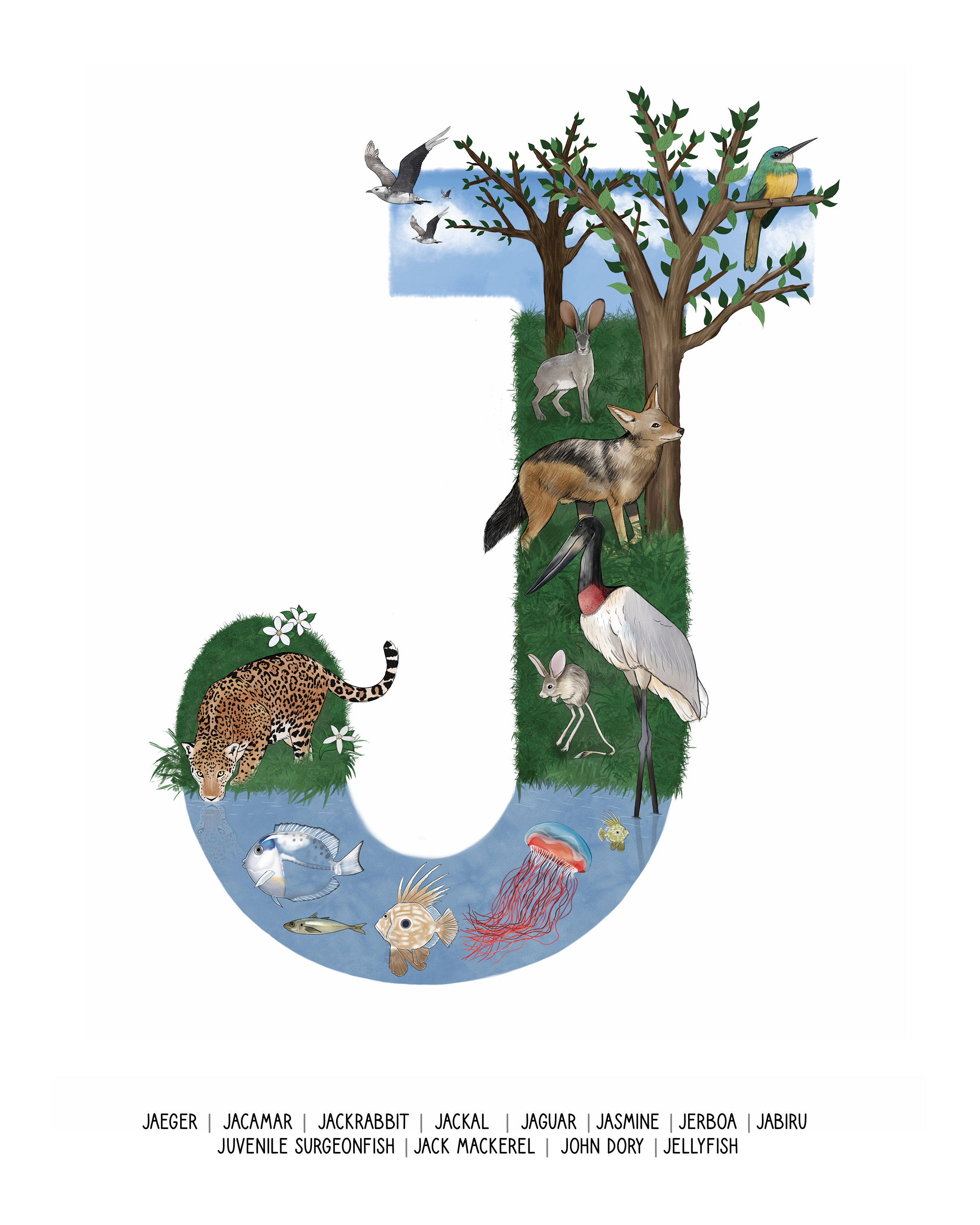The image showcases the letter 'J' set against a white background, artistically constituted by intricate nature illustrations. The top serif of the light blue letter 'J' features a view of the sky with birds flying, including one resting on a tree branch. Below, the scene transitions to land, displaying sprouting trees accompanied by various terraqueous animals: a jackal with prominent ears, a brown wolf with a black streak along its back, and a stork characterized by white feathers, a red-ringed neck, black head, and long beak. Near the stork is a distinctive jumping kangaroo mouse, featuring elongated legs, a long tail, large ears, and a small body. 

As the letter curves into its darker blue hook, the land morphs into an aquatic environment. Here, a vibrant collection of sea life includes a salmon-colored jellyfish, an octopus, a beige-colored fish, and possibly a whale. Emerging from the water and transitioning back to grassland at the base of the 'J', a leopard or jaguar is positioned, poking its head downwards. Around this area, various wooden animals are noticeable along with some brown and gray hues, completing the natural tableau.